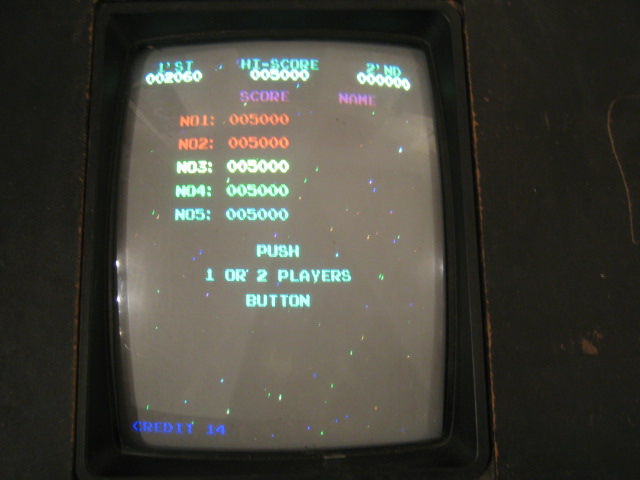The image features an old-fashioned CRT television screen, which is uniquely housed in a vertically oriented wooden casing. Displayed on the screen are details from an 80s-era video game. The screen prominently features green text instructing, "Push One or Two Players Button." Below this, a high score list is visible, though it appears unused, as all the scores are set at zero and no player names are listed. Subtly in the background, the screen shows a starry backdrop made of multicolored dots, suggesting that the video game might have an outer space theme, perhaps reminiscent of classic games like "Asteroids."